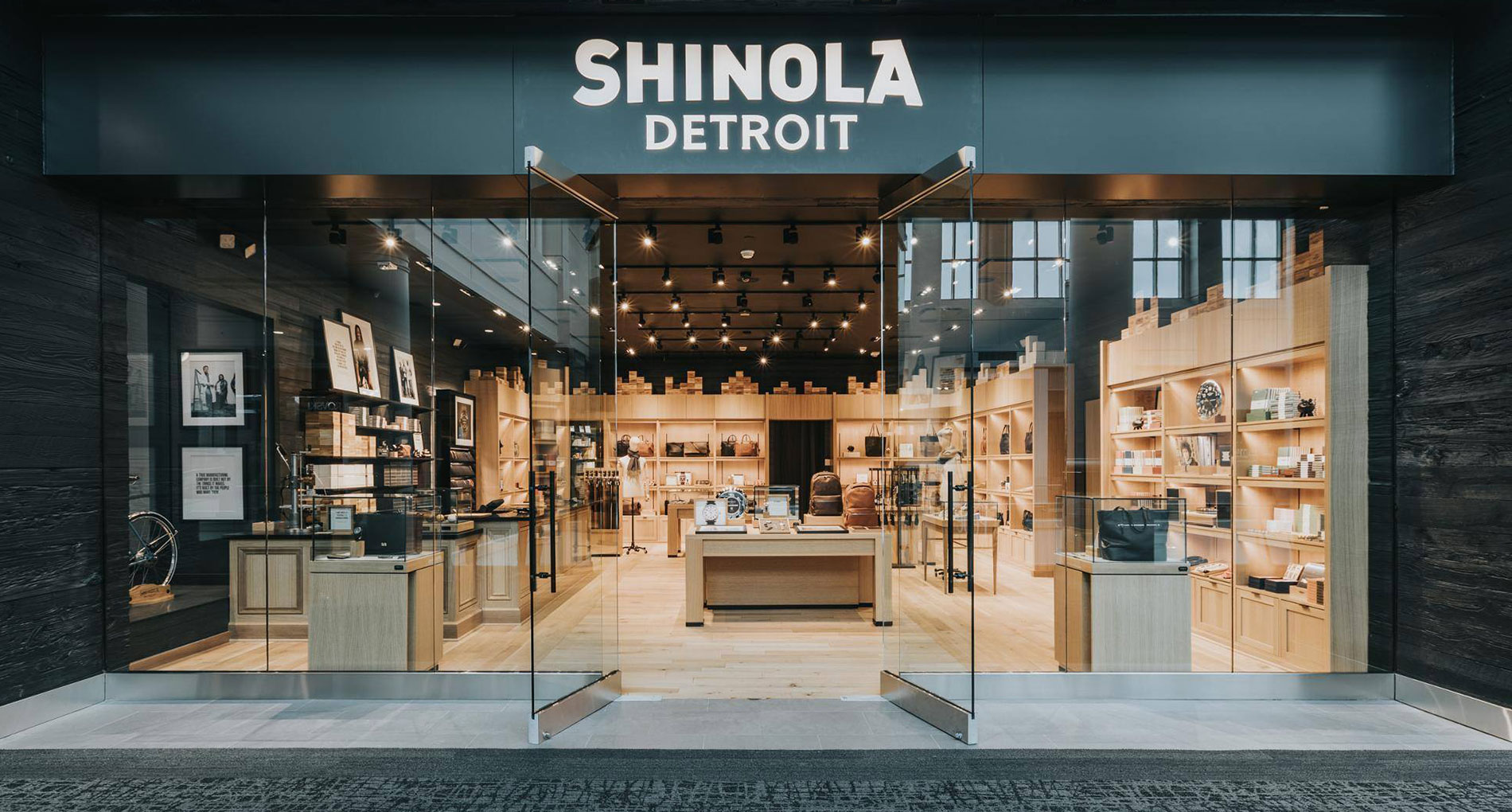This professional promotional photo captures an exterior view of a Shinola storefront. The storefront features glass doors centrally located and flanked by large glass windows, allowing a clear view of the interior. Above the entrance is a black rectangular sign with "Shinola" and "Detroit" written in white lettering. The left and right walls of the façade are painted black. The store is brightly lit, showcasing meticulously organized shelves with various shades of tan and brown, including a light brown feature wall adorned with items that may include framed photographs, home goods, and other merchandise. The color scheme prominently features black, white, gray, blue, and an array of tan and brown tones. Notably, there are no people in the image, emphasizing the store's design and layout for promotional purposes.